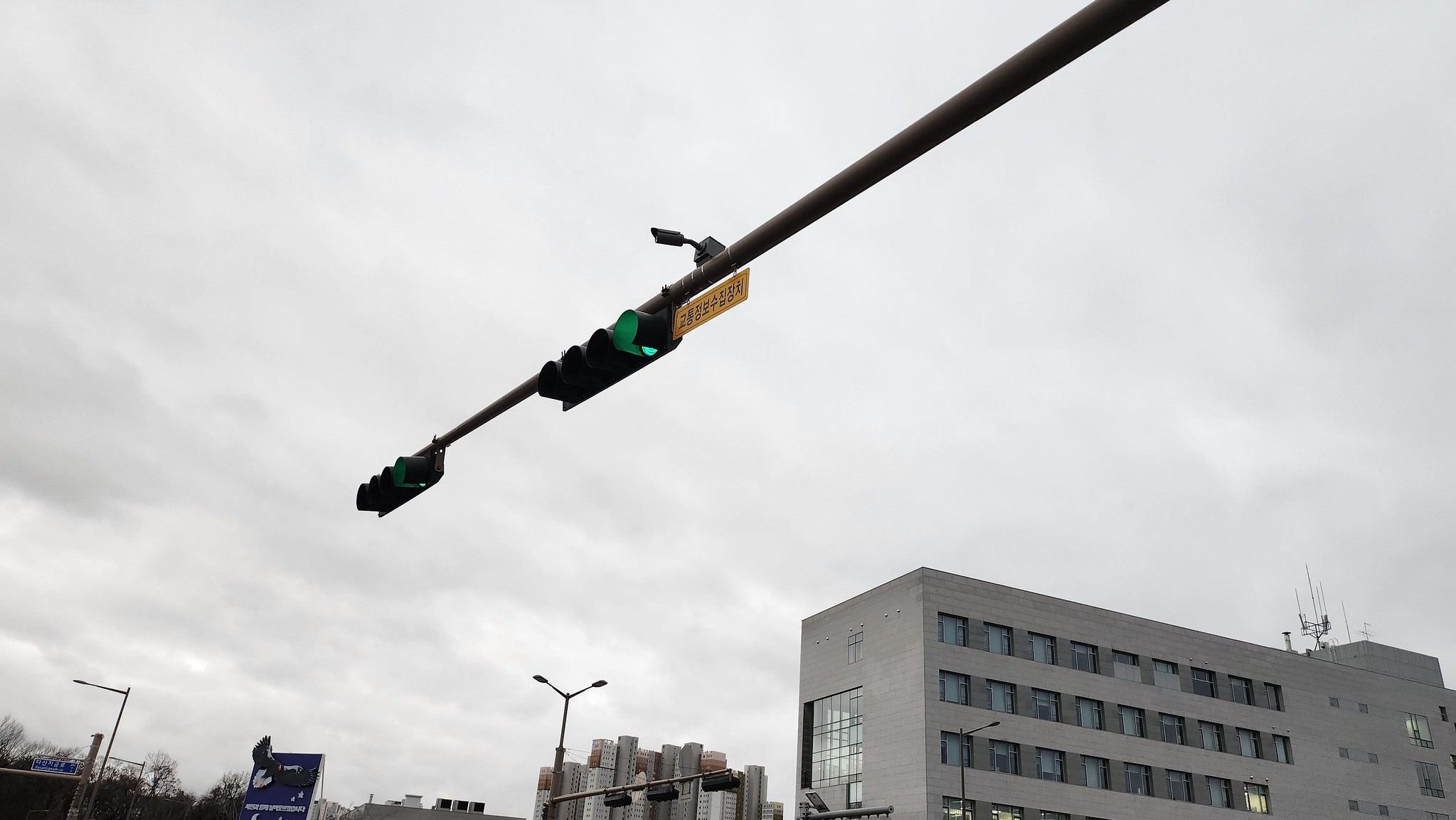The photograph captures a dynamic urban scene dominated by an overcast grey sky. Central to the image is a large black pole supporting two sets of traffic lights, each with four lights. Both sets of traffic lights show green, visible from the ground perspective looking upwards. Suspended from the pole is a yellow sign and a small security camera. In the background, a variety of buildings are visible, including a dull grey concrete brick building with numerous windows, likely around 30. Further back, high-rise flats dot the skyline, suggesting a densely populated area. Two additional streetlights and a purple billboard, difficult to decipher but likely written in Korean, hint at the location's vibrant yet slightly dreary urban character.